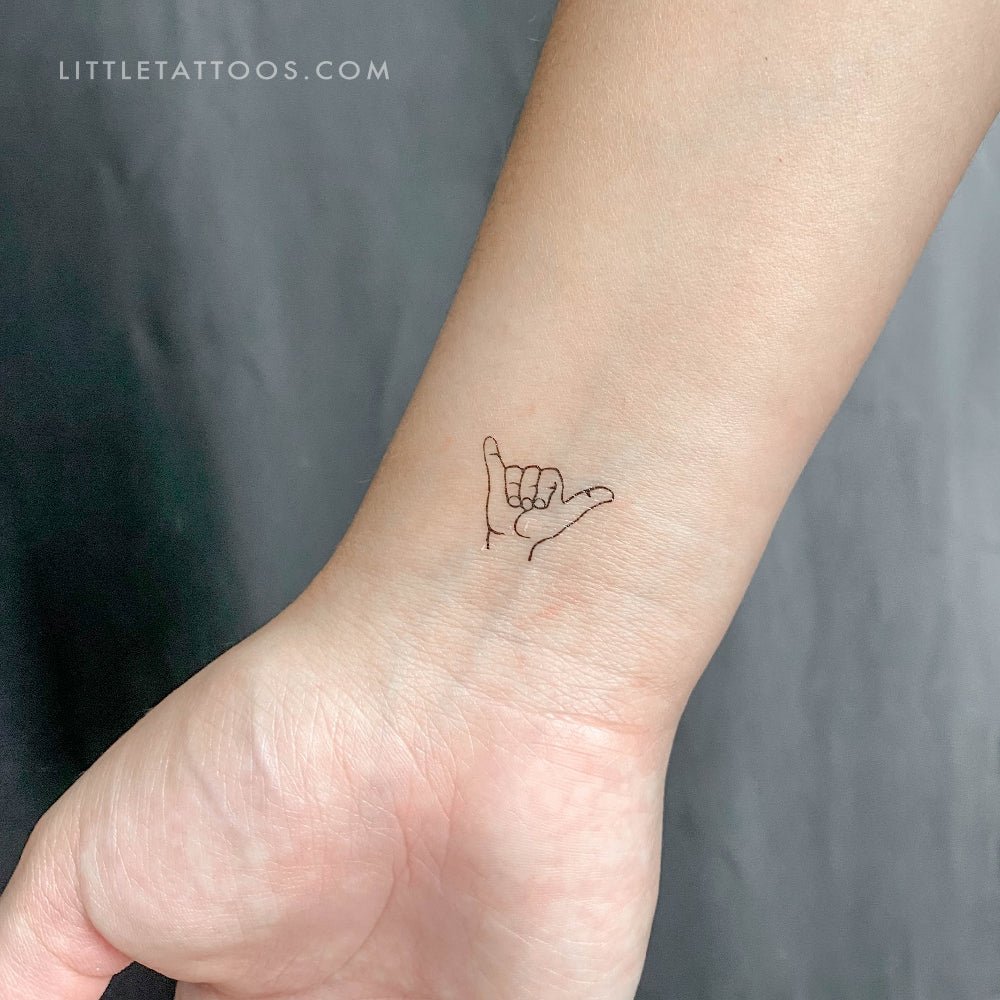In this image, we see a person's wrist and a portion of their forearm and palm, with a faint black ink tattoo prominently displayed. The tattoo depicts a hand with three middle fingers — the index, middle, and ring fingers — bent downwards, while the thumb and pinky extend outward, resembling a hand signal. The person appears to have light, possibly Caucasian skin. The background of the image is a plain gray color. In the upper left corner of the image, the text "LITTLETATTOOS.COM" is printed in white, uppercase letters.